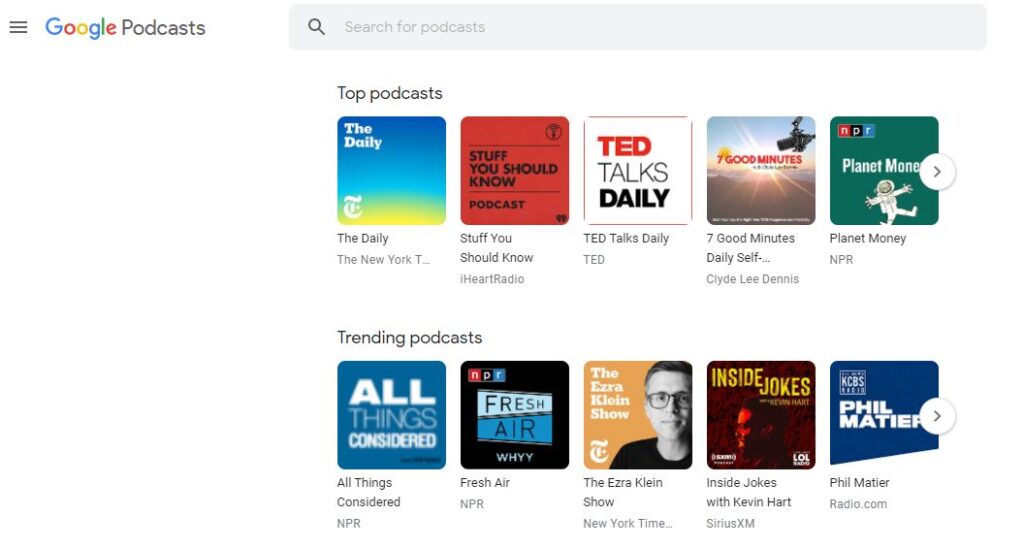This image is a detailed screenshot of a computer displaying the Google Podcasts interface. In the upper-left corner, there is a three-line icon (often referred to as the hamburger menu), adjacent to the "Google Podcasts" label. To the right of this, there is a gray search bar.

The interface is divided into two sections: "Top Podcasts" and "Trending Podcasts." 

In the "Top Podcasts" section, there are five highlighted podcasts:
1. **The Daily**: Featured with a blue and yellow square above it.
2. **Stuff You Know**: Displayed in red with black font.
3. **Ted Talks Daily**: Also in red and black font.
4. **Seven Good Minutes**: Showcasing an image of a skateboarder mid-air.
5. **Planet Monday**: Highlighted with a green square and features a white figure with arms and legs outstretched.

Below, the "Trending Podcasts" section lists the following shows:
1. **All Things Considered**: Presented with a blue square labeled "All Things Considered."
2. **Fresh Air**: Featured with a light blue and darker blue square bearing the words "Fresh Air."
3. **The Ezra Klein Show**: Displaying an image of a male wearing glasses and a black shirt.
4. **Inside Jokes with Kevin Hart**: Showcased with a brown square and an image of a Black man.
5. **Phil Mater**: Highlighted with a blue square labeled "Phil Mater."

Each podcast is visually represented with distinctive colors and images, making the interface visually appealing and user-friendly.